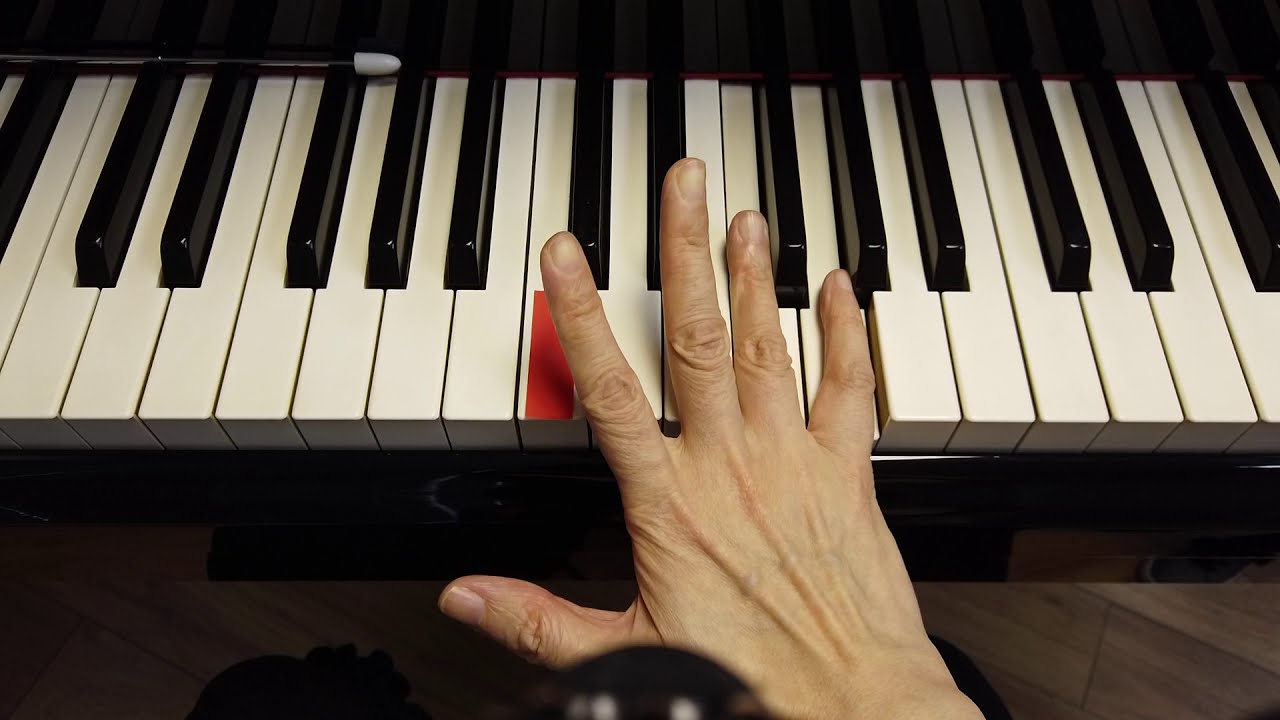This color photograph, resembling a freeze-frame from a video, depicts a detailed top-down view of a piano keyboard. The scene is centered around an older woman's hand with short nails, her fingers slightly crooked, delicately positioned over the keys. Her tiny pinky finger and the adjacent fourth finger are pressing down on white keys, while her index finger points towards a key marked distinctively with a wide, reddish-orange rectangular tape. The photo captures the black and white keys of the piano extending horizontally across the frame. Behind the keys, in the upper left corner, a conductor's baton with a white tip rests. The shiny black surface of the piano case edges into the scene, and just below the keyboard, a glimpse of wooden flooring and a couple of foot pedals can be noted. The image exudes a high-quality, realistic, and photographic style, devoid of any text.